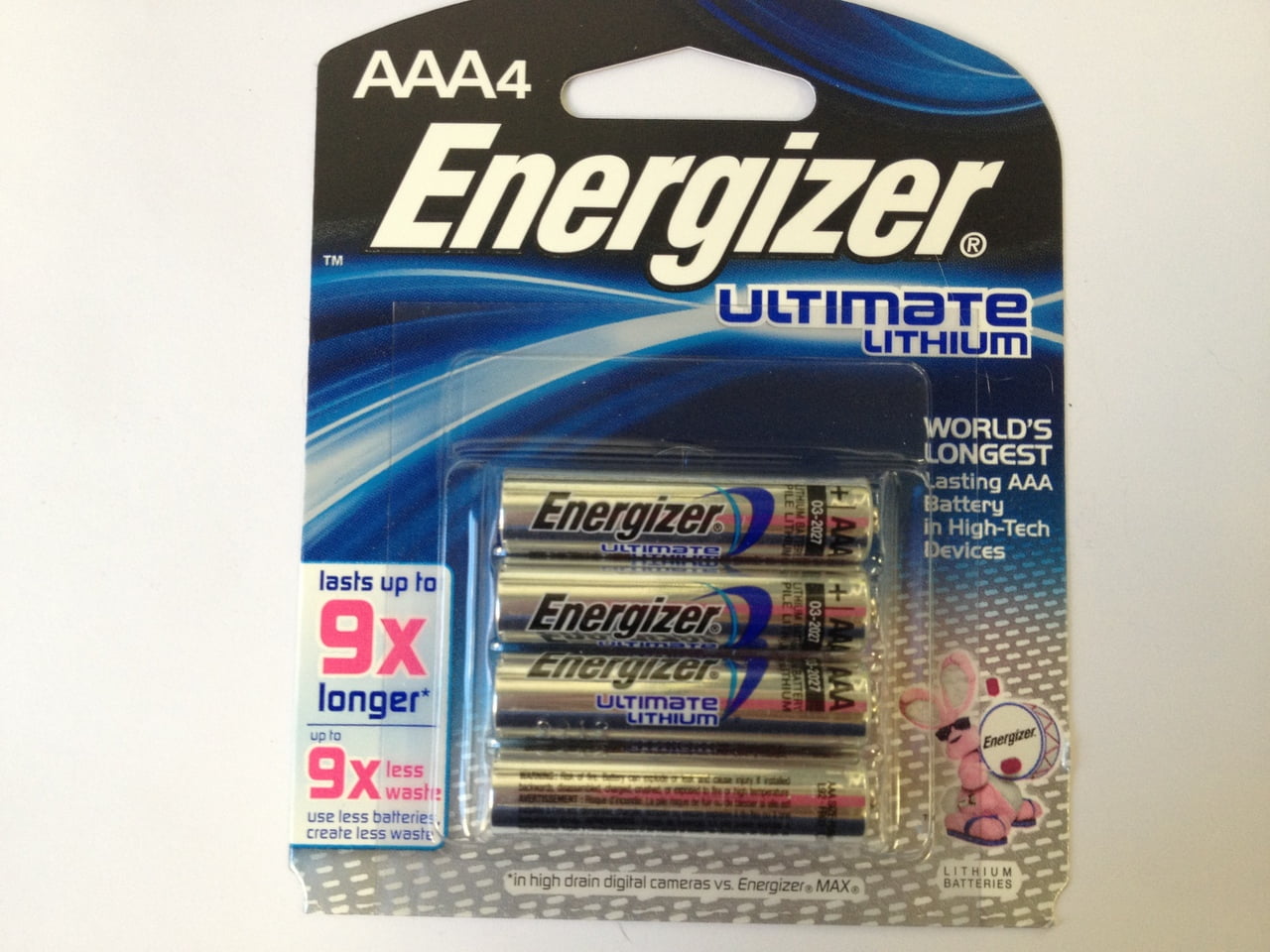This photograph displays a neatly sealed pack of Energizer AAA batteries. The package prominently features the branding at the top left corner, where "AAAA4" and "AAA4" are printed. The top section of the package has a black background with "Energizer" emblazoned in bold white letters. Below this, on the right-hand side, the text "Ultimate Lithium" is accompanied by dynamic blue energy streaks, adding a touch of high energy to the design. 

Encased within clear, see-through plastic, the AAA batteries are visibly secured and well-arranged. To the right of the batteries, there's a bold claim that reads, "World's Longest Lasting AAA Battery in high-tech devices." Additionally, the iconic pink Energizer bunny is positioned below this text, reinforcing the brand's identity. The overall appearance of the packaging conveys a message of long-lasting power and advanced technology.